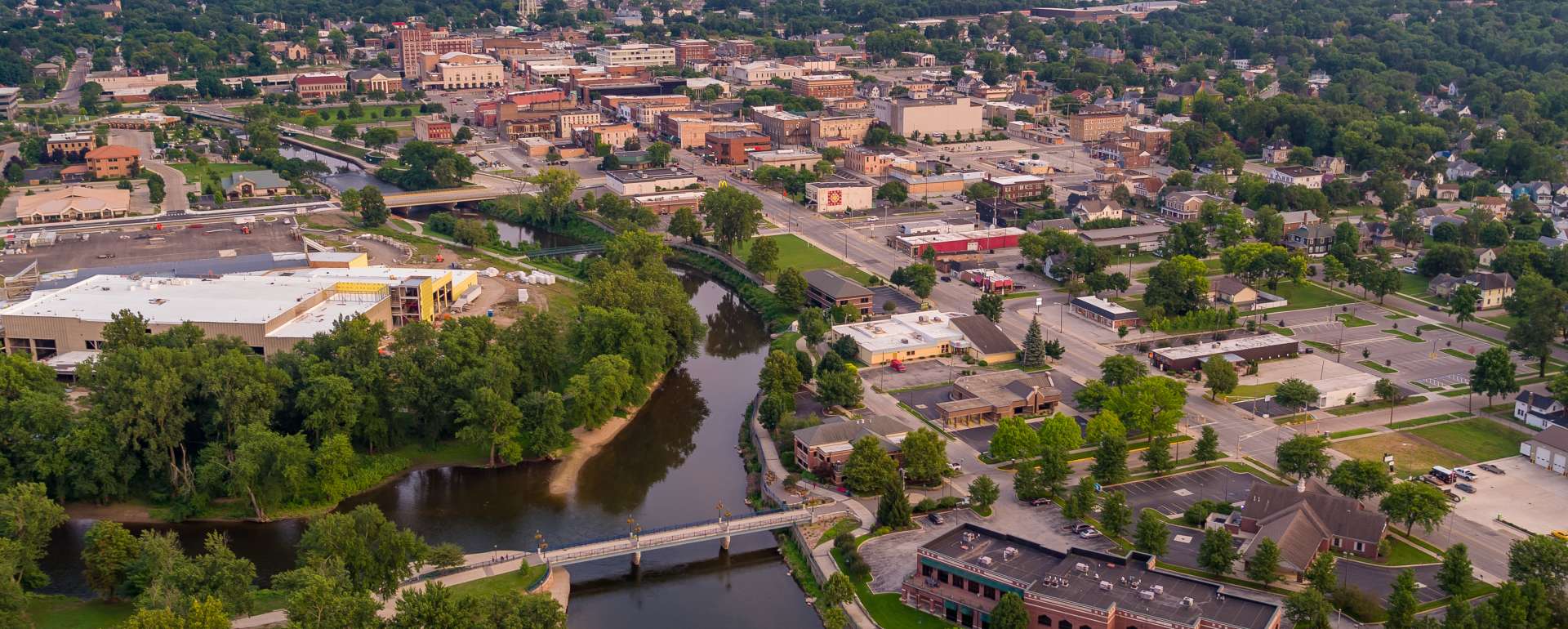The aerial photograph showcases an expansive view of a city, featuring a mix of natural and urban elements. At the heart of the city, a river flows predominantly vertically, with a canal diverging in the lower left section. Several bridges span the river, notably one near the bottom and another towards the top. The left side of the image is dominated by a significant building enveloped in greenery, while the right side is more densely packed with a variety of structures and main roads. The cityscape is a blend of rooftops, parking lots, and paved streets surrounded by an abundance of trees, both planted and wild, indicating well-thought-out urban planning. The upper sections of the photograph reveal the city's connection to larger wooded areas. Despite the numerous roads, the image captures a tranquil moment with few cars in sight, suggesting a quieter time of day.